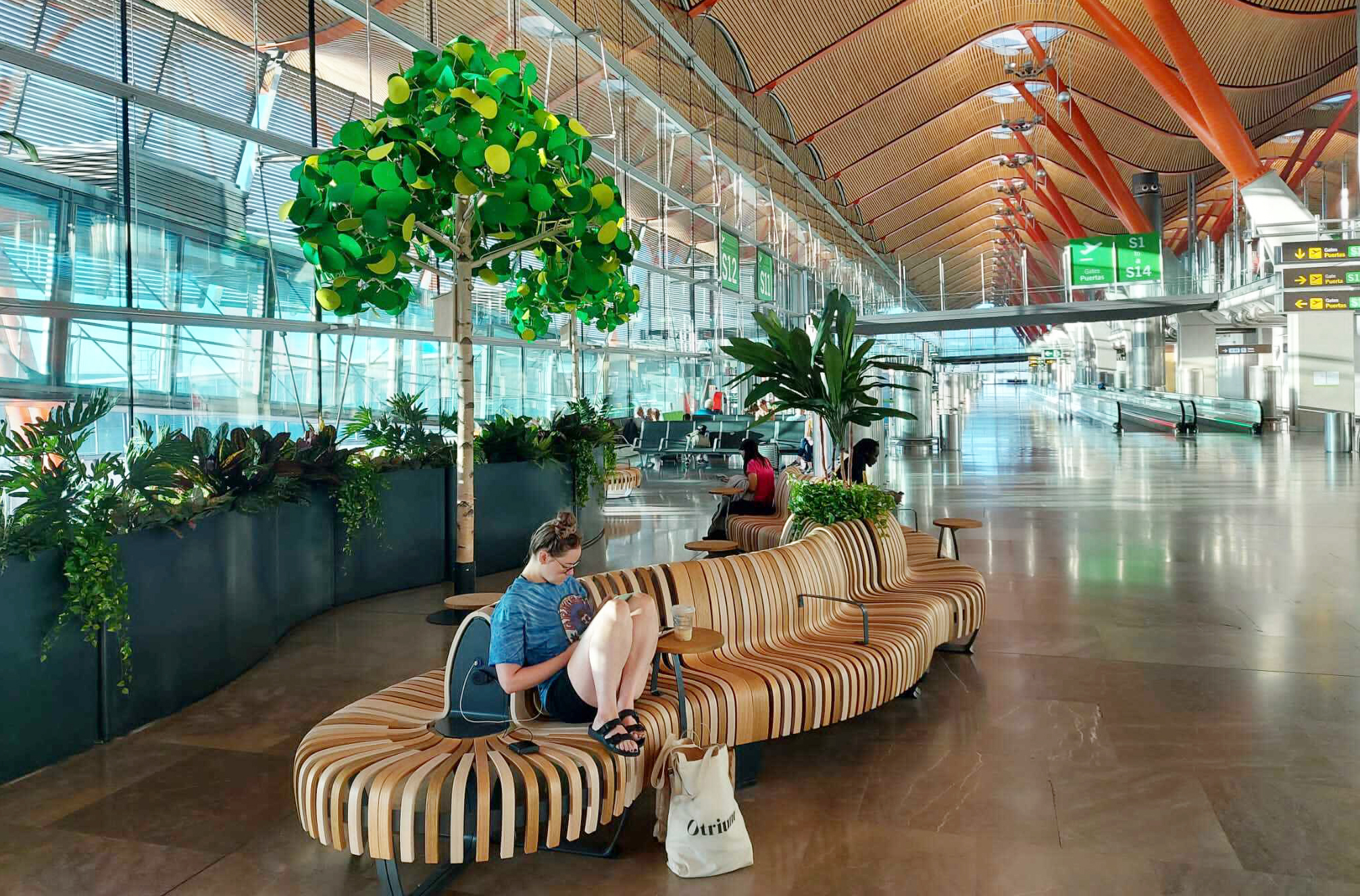The image depicts a spacious, well-lit area that appears to be an airport. Dominated by large windows, the room is flooded with natural light, highlighting the brown marble tile flooring and the high, peaked ceiling supported by prominent red beams. The right side features an array of large green plants, including a tree housed in a black retaining wall with additional plants cascading over it. Further back, the room is sectioned off, leading to various parts of the airport. 

In the center of the image, a woman sits comfortably on a uniquely designed wooden bench with artistic curves and a wavy structure. The woman, with her hair tied up in a bun, is wearing glasses, a blue tie-dye shirt, black shorts, and black sandals with her feet casually placed on the bench. A canvas bag lies at her feet, and she appears to be engrossed in reading a book. The setting's ambiance is both serene and sophisticated, marked by the blend of modern architectural elements and lush greenery. Additionally, directional signs in green and yellow with white text are visible in the background, hinting at the navigational aids typical of an airport environment.